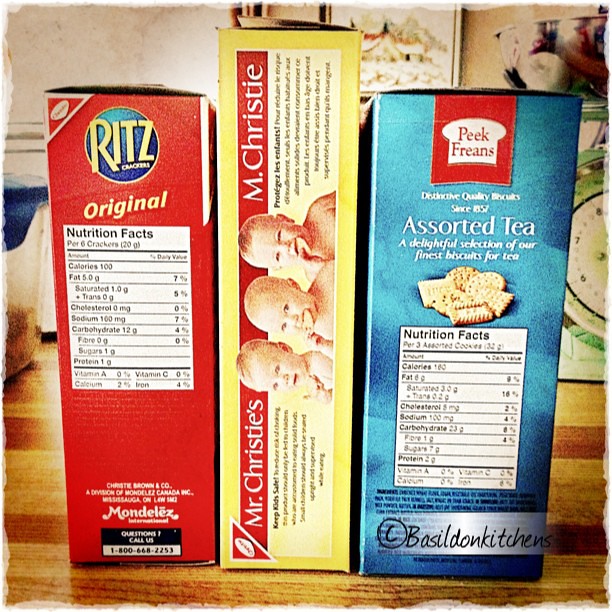The image showcases an assortment of three cracker boxes arranged on a wooden kitchen countertop, with a copyright watermark for Basil Dawn Kitchens. On the left, the red box of Ritz original crackers prominently displays its nutritional facts, including 100 calories per 6 crackers, and contact information (1-800-668-2253). In the center, Mr. Christie's crackers feature an illustration of three babies, each enjoying a cookie, but no nutritional information is visible on this box. To the right, a blue box labeled Peek Freans contains assorted tea crackers, with nutritional facts partially shown. The background reveals a kitchen setting with a scale and a bowl, likely Tupperware storage, and possible artwork on the wall.